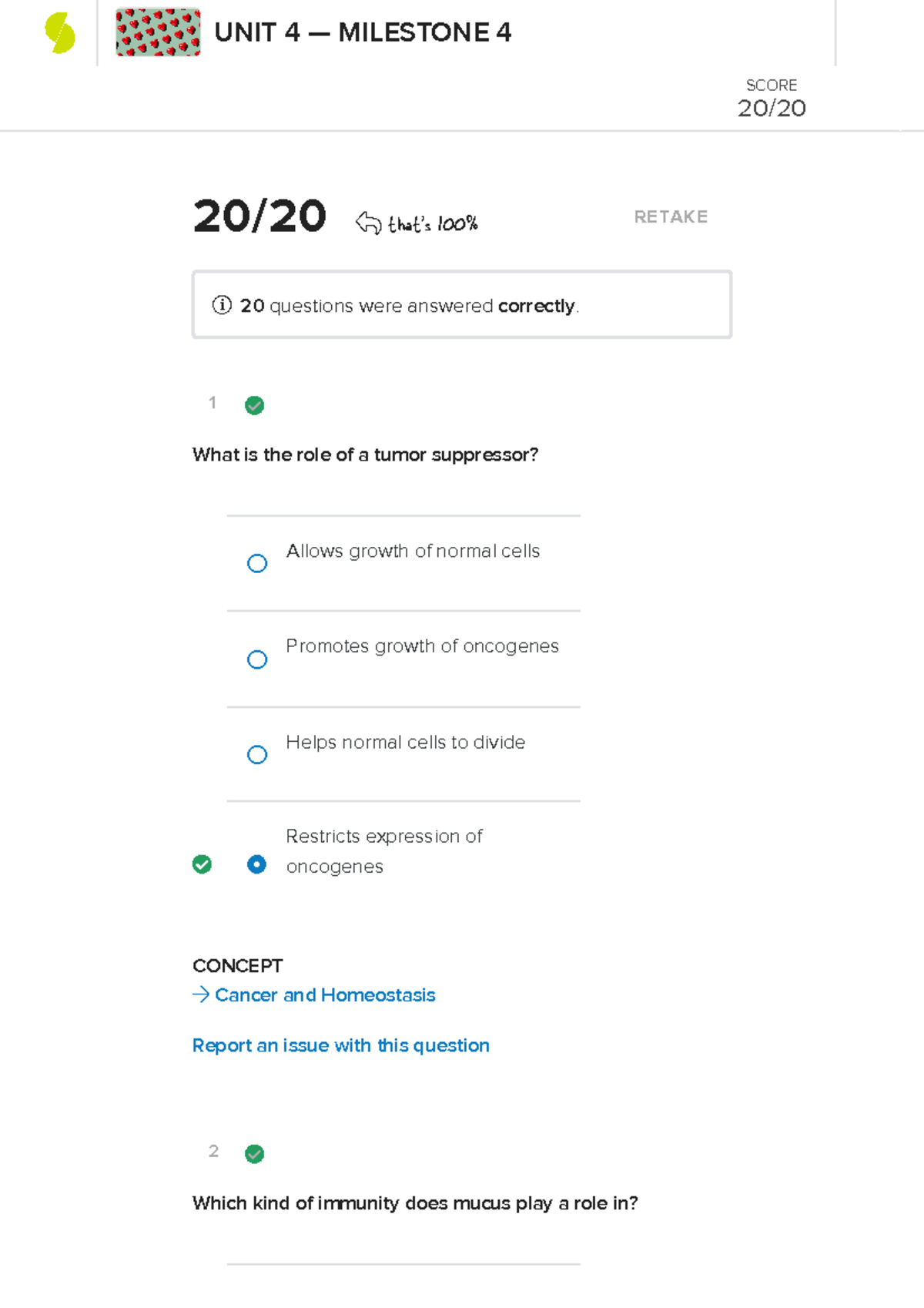The image features an educational interface with a variety of detailed components. The background is white, and the top of the image prominently displays the heading "Unit 4 Milestone 4." To the left of this heading, there is a lightly green square adorned with red hearts arranged in a list format. 

Further to the left of the green square, there is a logo consisting of a green circle bisected by a horizontal line, resembling the letter "S." On the top-right corner of the image, the text "Goal 20 of 20" is displayed.

Below the top section, the main page contains black text that reads "20 of 20" followed by "100," indicating a perfect score. The option to "Retake" is also visible. The caption notes that 20 questions were answered correctly.

The first question displayed is: "What is the role of a tumor suppressor?" with the possible answers being:
- Allows growth of normal cells.
- Promotes growth of oncogenes.
- Helps normal cells divide.
- Restrict expression of oncogenes.

The selected answer, "Restrict expression of oncogenes," is marked with a green tick, signifying it as the correct choice.

Beneath the first question, there is a section labeled "Concept," divided into two parts with the topics "Cancer" and "Homeostasis" written in blue text. Additional text mentions "Reports and issues with this question."

The second question on the list is also indicated as correct. It asks: "What kind of immunity does mucus play a role in," though the possible answers are not shown.

Overall, the image reveals a multiple-choice interface where the user has answered all 20 questions correctly, earning a score of 100%.